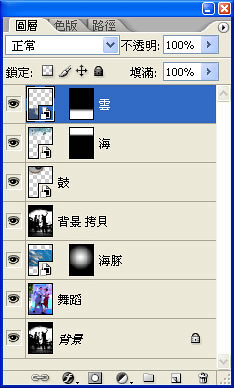The image is a detailed screenshot of an old graphic editing program, likely running on Windows XP or an even older version of Windows, as indicated by the dark blue borders and vintage window control icons for minimizing and exiting. The user interface displays the layers section, which resembles a table comprising various rectangular areas with different symbols, indicating the contents of each layer. Text throughout the image is primarily in Japanese or Chinese kanji, adding to the visual complexity.

On the left side of the layers panel, there are icons representing functions such as visibility (eye symbols) and layer locking (padlocks). Notable visual elements include images within layers: some in color, such as a man in a blue suit and a woman in a red skirt, appearing to be singing or dancing, and other black and white illustrations. Checkerboard patterns of white and gray indicate transparent areas.

Additional interface elements include arrows for navigation, the zoom level indicated twice as 100%, and a scroll bar on the right for vertical navigation. At the bottom, there are multiple action icons, including a chain, Facebook logo, square with a circle inside, yin-yang symbol, folder, piece of paper, and a bin. Intricate details of colors such as light blue, dark blue, black, tan, gray, and purple populate various squares and lines, including bar graph-like structures, making the overall layout visually rich and complex.